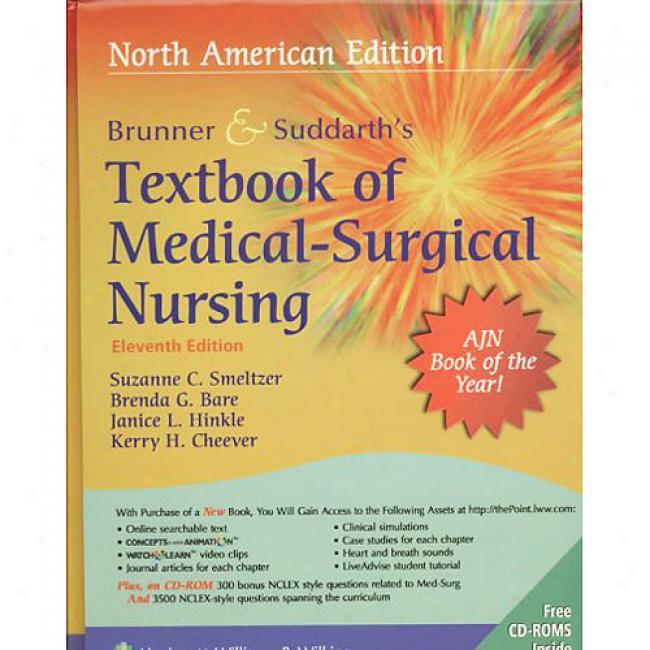The cover of Brunner and Suddarth's "Textbook of Medical-Surgical Nursing," North American Edition, 11th edition, features a vibrant yellow and orange background with a large, starburst design in orange on the upper right side. Prominently displayed in the starburst is a red circle containing a sun-like graphic formed by numerous triangles, emblazoned with "AJN Book of the Year!" in bold text. At the top, white lettering announces "North American Edition," with a white line running below it. The title, "Brunner and Suddarth's Textbook of Medical-Surgical Nursing," is prominently written, followed by the names of the authors: Suzanne C. Smeltzer, Brenda G. Bare, Janice L. Hinkle, and Kerry H. Cheever. Detailed information about the included assets mentions that with the purchase of the new book, readers will gain access to additional resources, and a note in the lower right corner highlights that free CD-ROMs are included.